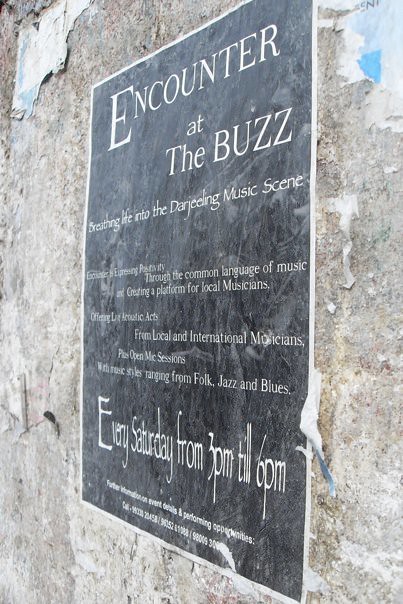The image depicts a black, weathered sign affixed to a severely weathered gray stone wall with peeling paint. The sign is positioned at an angle, making some text difficult to decipher. The prominently displayed white text reads, "Encounter at the Buzz," followed by, "Breathing life into the Darjeeling music scene." Beneath this, smaller text states, "Through the common language of music," and mentions a platform for local musicians, inclusive of both local and international talent. It highlights live acoustic performances, including open mic sessions, with genres ranging from folk to jazz and blues. Larger text towards the bottom announces, "Every Saturday from 3 p.m. till 6 p.m." Finally, there is very fine print at the bottom, which seems to provide contact information, although it is too faded to read clearly.